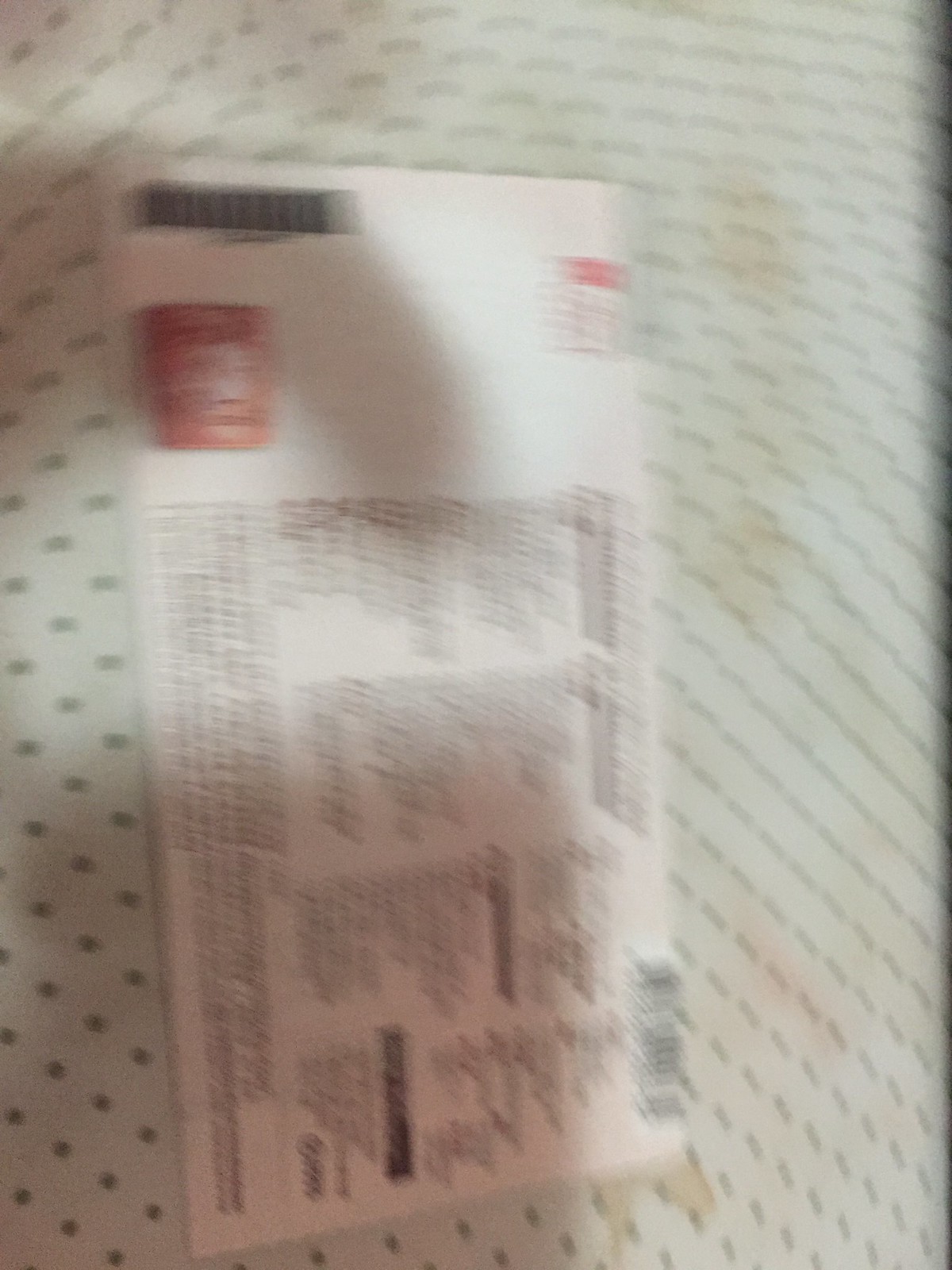A blurry photograph captures a rectangular piece of paper resting on a white platform adorned with gray polka dots. The paper itself is difficult to read due to the blurriness and the small size of the text, which requires tilting the head to the right for proper orientation. At the top left of the paper, a distinct black bar is visible, followed by a red logo directly beneath it. Below the logo, there are several paragraphs of extremely small, sideways text. In the bottom right corner, a barcode can be discerned. The background of the image, similar to the platform, features a white surface with evenly distributed gray polka dots.